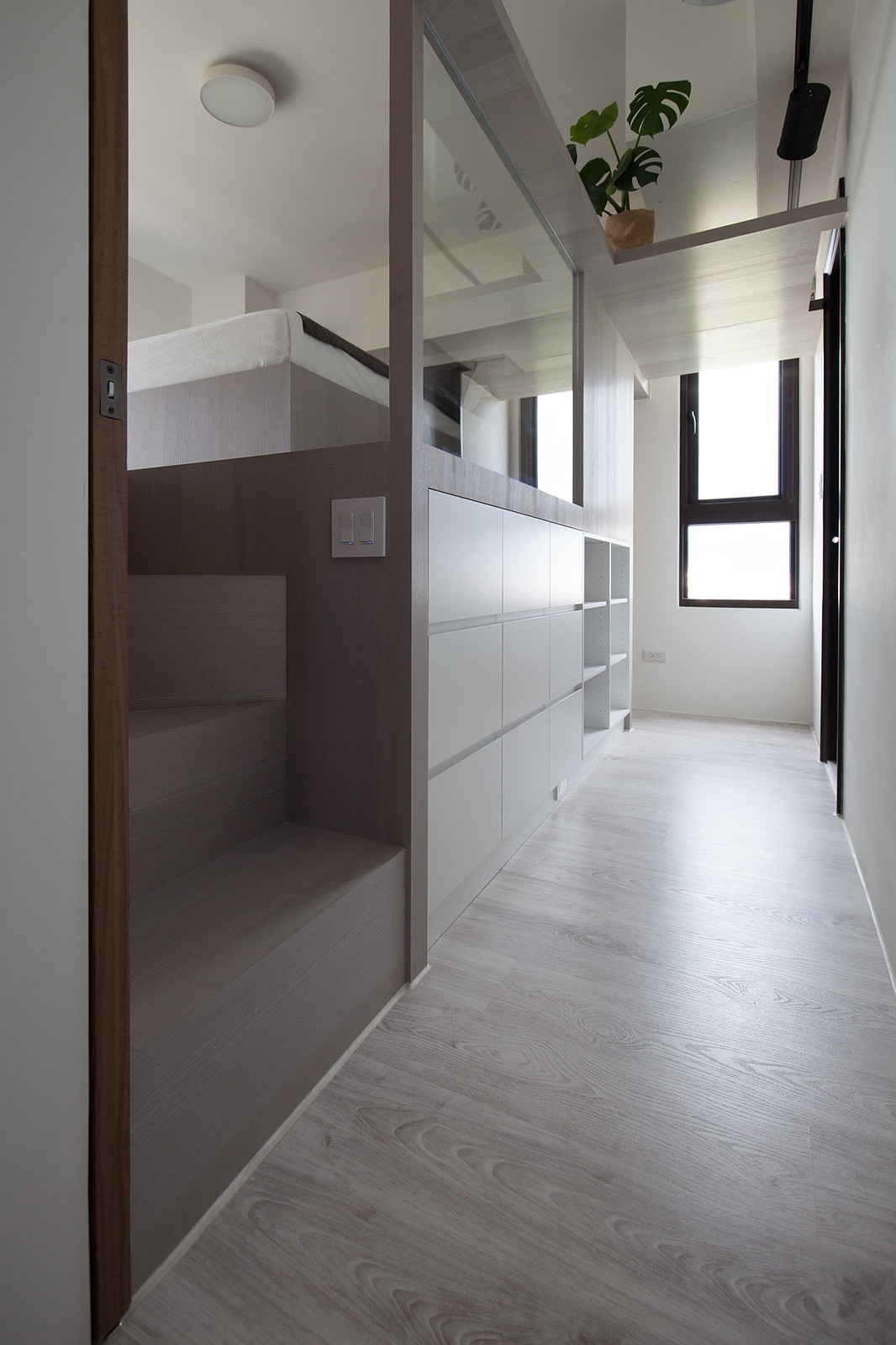This image depicts a vertically oriented hallway in a house, characterized by its neutral color palette of grays, whites, and blacks, which gives it a monochromatic yet modern appearance. The hallway floor is finished in a gray wood look, featuring visible wood grain patterns. On the left side, immediately at the start, there is a gray stairwell with the first two steps visible, leading up to a higher living area. The adjacent wall to the stairwell is gray with lighter gray square panels arranged in horizontal rows, ultimately transitioning into a three-shelf unit at the end.

To the right, a flat gray wall extends the length of the hallway. As the hallway progresses, a black-trimmed doorway appears on the right side, with a window at the hallway's end. This window, set against a white wall, is framed in black and appears to be potentially open. Above, the ceiling mirrors the gray flooring, creating a cohesive look with a strip of this flooring extending down the left side and widening out as it reaches the shelving unit, connecting the ceiling to the left wall.

A potted plant in a brown wicker pot with large green leaves adds a touch of color and life, positioned atop the shelving section near the end of the hallway. The monochromatic theme extends to the window frames and the door edges, creating a refined and thematic visual effect. The brightness outside the window adds contrast to the subdued interior tones.